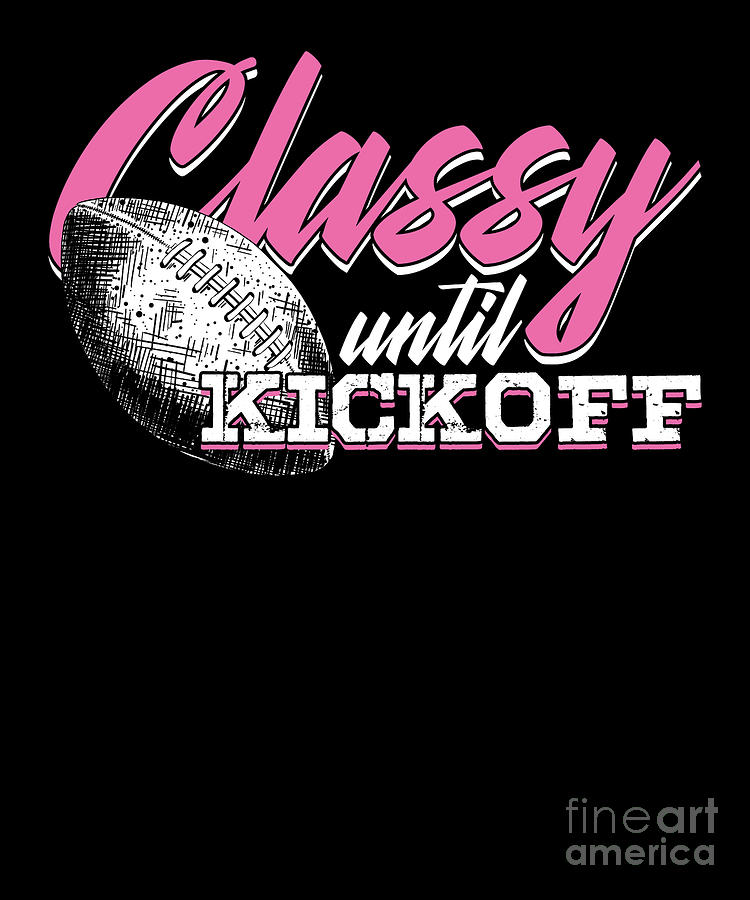This image is an advertisement for an event titled "Classy Until Kickoff." The entire background is solid black, creating a striking contrast with the text and graphic elements. At the top center, the word "Classy" is rendered in a pink script font, outlined in white, giving it a refined yet bold appearance. Directly beneath, the word "Until" is displayed in a free-flowing white font that matches the elegance of the word "Classy." Below that, the word "Kickoff" stands out in an all-caps white font with a pink drop shadow, making it eye-catching against the dark background.

To the left of the text, there's an intricate pen-and-ink drawing of an American football. This football is primarily black and white with detailed stitching, partially overlaying the letter "C" in "Classy" and appearing behind the word "Kickoff." The bottom right corner of the image features a grey watermark that reads "Fine Art America," with the words "Fine Art" positioned above "America." The overall design suggests a classy-themed football event, blending elegance with the rugged imagery of the sport.